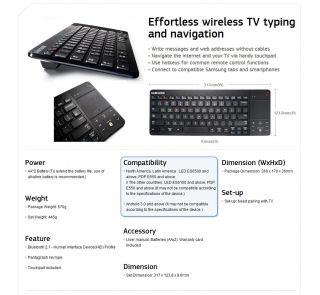This image is a detailed screenshot from a website that predominantly features a wireless keyboard. The background is clean and white, allowing the various elements to stand out clearly. On the left side, there are two separate images of the keyboard, each showcasing different angles. 

The image at the top gives a side view of the keyboard, highlighting its slim profile that extends subtly towards the back. The lower image provides a close-up of the right section of the keyboard, capturing its detail accurately.

Overlaying these images is a bold headline in blurred print that reads, "EFFORTLESS WIRELESS TV TYPING AND NAVIGATION". Beneath the headline are several bullet points, but the text is obscured and not legible.

Continuing downward, the webpage lists the dimensions of the keyboard and displays an image of the keyboard itself. The keyboard is black with distinct white lettering and numbers on its keys.

Further down, there is a section divided into squares. One square, with a pale blue background, is labeled "Compatibility" although the text within this section is also blurred and pale. Another square contains information on "Power," "Weight," and "Features," but again, the text inside remains blurry.

Lastly, the image includes sections titled "Accessory Dimension" and "Setup." To the far right, there is a mention of "Dimension" with a specification in parentheses stating (W x H x D), which translates to Width times Height times Depth. The exact details in these sections are unclear due to blurring.

Overall, the image effectively showcases the main features and technical aspects of the wireless keyboard, despite some text being blurred.